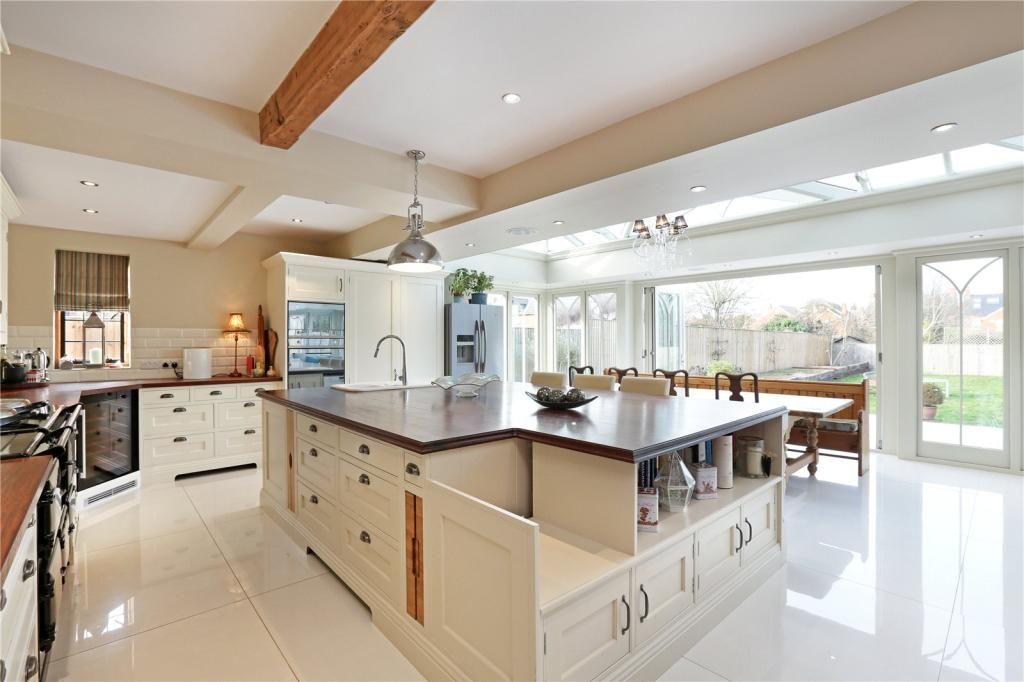This image captures the interior of a spacious and modern kitchen inside a home. Dominating the center is a significant island with a black top and light wood base, incorporating a built-in sink and various storage drawers, including some slide-out shelves and sections with handles. The island also features spaces adorned with decorative items such as flower pots and jars. To the right of the island stands a long dining table with four brown chairs, offering a view through wide glass doors that lead out to a grassy backyard. The kitchen's floors are covered in white marble tile, complementing the white ceiling. 

On the left side of the kitchen, there's a main cooking area complete with a gas burner stove and a backsplash window above a brown countertop. The kitchen appliances include a gray refrigerator topped with flower pots, and another refrigerator with a glass door is noted on the left. Above the island, and near the entrance to the backyard, hang modern lighting fixtures that illuminate the space. The room features a mix of open shelves and cabinetry, particularly white shelving around another steel appliance which may include ovens or additional storage. The modern design is accentuated by a molded ceiling and a distinctive wooden beam running from the center towards the lower part of the kitchen, effectively intertwining the contemporary elements with a touch of warmth from the wood accents.